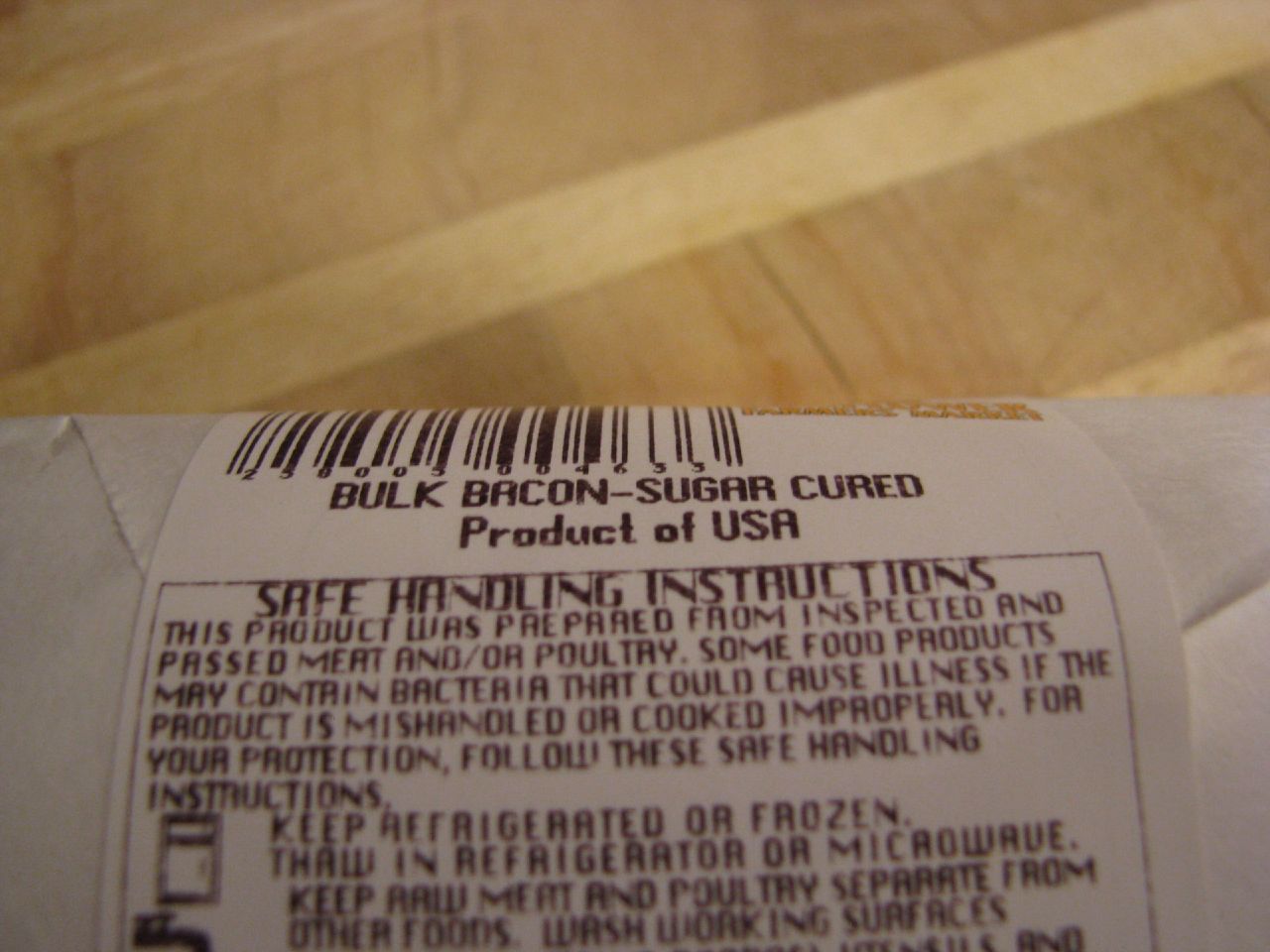The image showcases a neatly packaged product placed on a light brown wooden floor characterized by thin wooden strips running horizontally. Occupying the lower half of the image is a white label wrapped around the package, which itself appears to be encased in white wrapping paper. The top part of the label features the text "Bacon" in bold black letters, followed by "Sugar Cured" and "Product of USA." Below this, there is a black box containing safe handling instructions and information about how the product was prepared from inspected and passed meat and/or poultry, along with storage guidelines. The detailed packaging and labeling ensure clarity and safety for consumers.